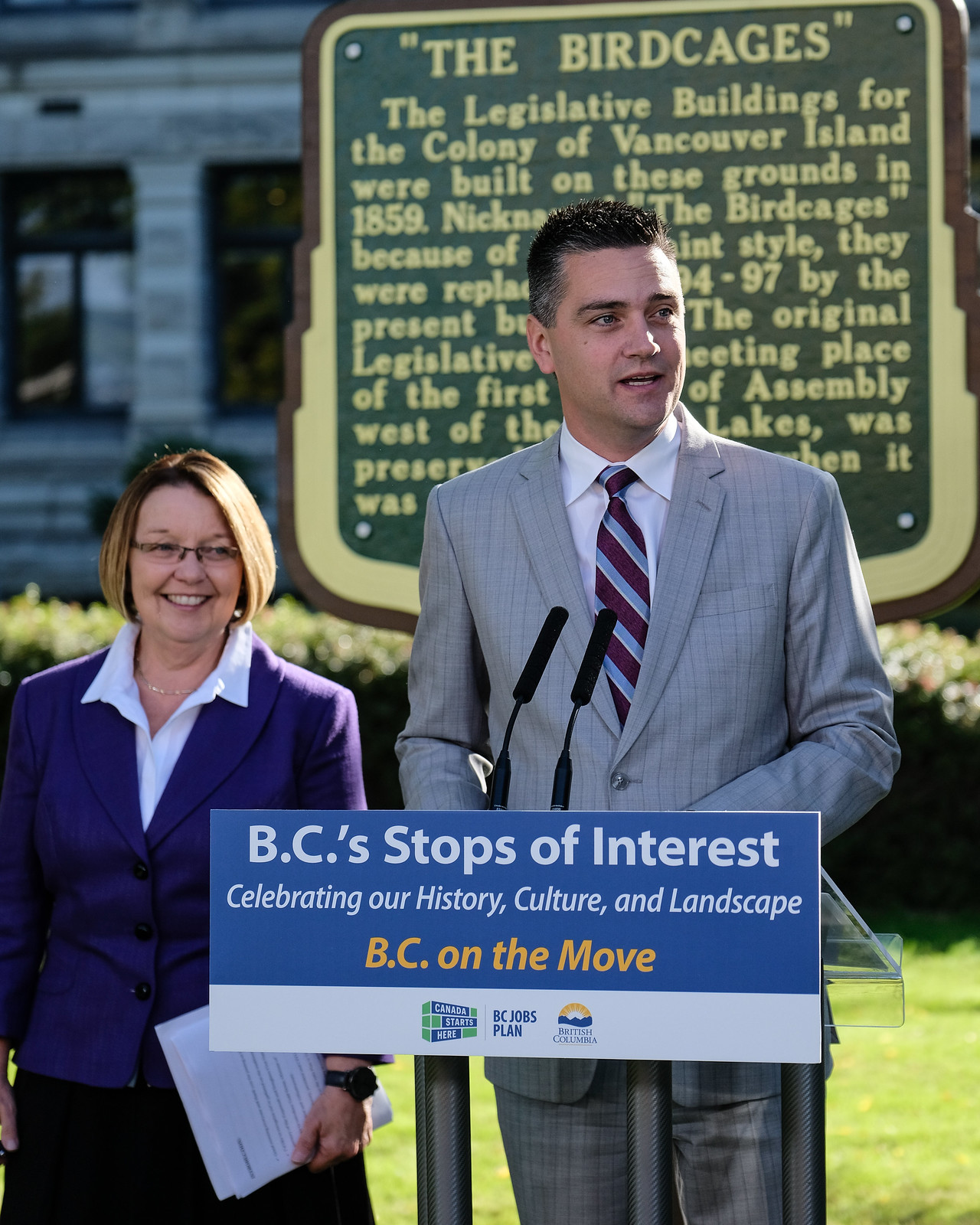In the photograph, taken outdoors, a man and a woman are standing behind a clear acrylic podium with a blue and white placard that reads, "BC Stops of Interest: Celebrating Our History, Culture, and Landscape". Below this, in yellow text, is written "BC On the Move". The sign also features the logos "Canada Starts Here", "BC Jobs Plan", and "British Columbia" at the bottom. The man in the foreground is wearing a gray suit with pinstripes, a white undershirt, and a multi-colored striped tie comprising black, white, yellow, and blue stripes. He stands facing the podium but looks to his right. In front of him on the podium are two black microphones. To his left, a woman is dressed in a blue button-up jacket over a white blouse and a black skirt, holding several papers. Behind them, a large green sign with a brown border and yellow text outlines historical information, reading "The Bird Cages" and detailing the legislative buildings built in 1859 on the grounds of the colony of Vancouver Island.